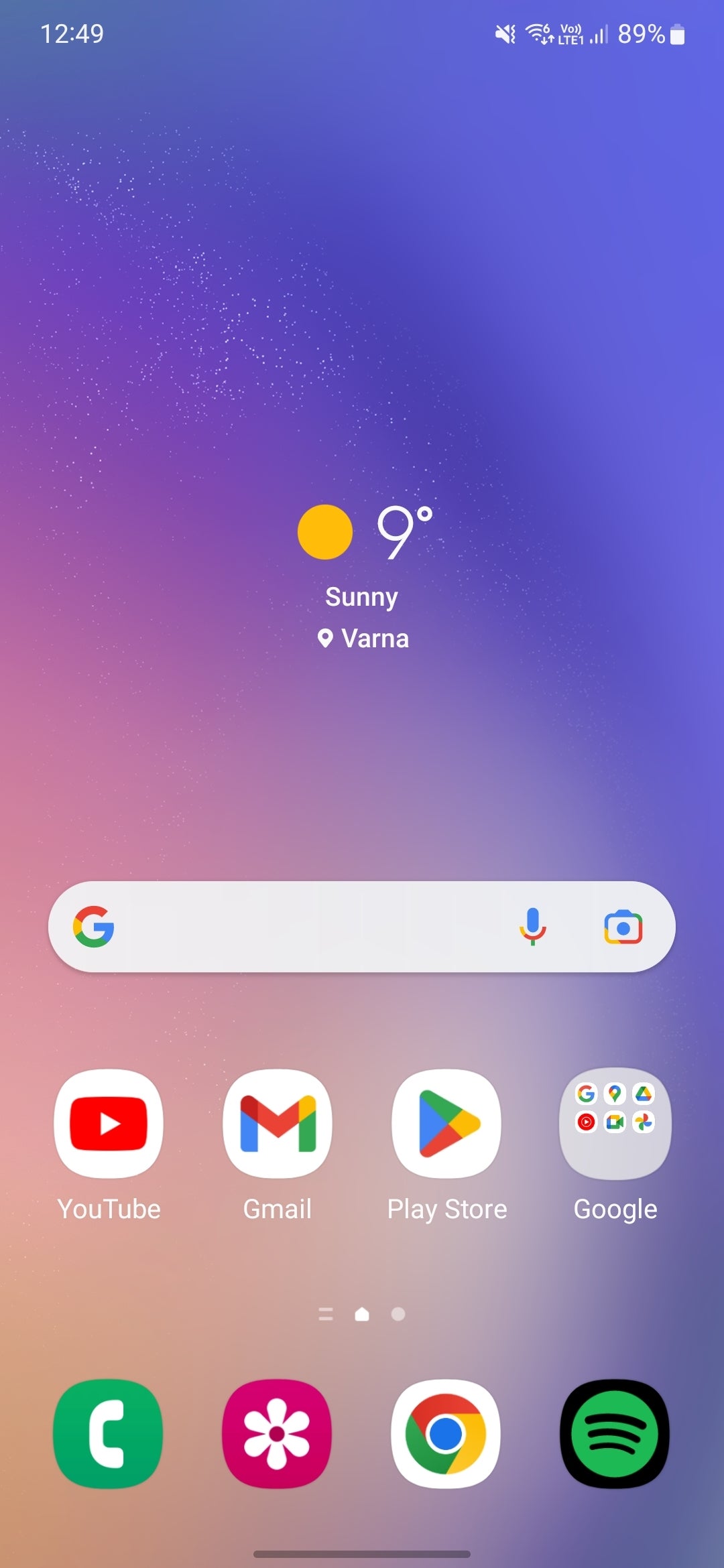This image depicts the home screen of an Android phone. The wallpaper features a gradient background with a blend of blue and purple hues in the top-right corner and orange and yellow tones in the bottom-left corner, creating a diagonal transition of colors. 

At the top-left corner of the screen, the time is displayed as 12:49. On the top-right corner, various status icons are shown, including a battery icon indicating 89% charge, a Wi-Fi 6 icon, a mute icon, and a signal icon labeled VOLTE1.

Centrally positioned on the home screen, there is a yellow circle representing the sun; the weather is shown as sunny with a temperature of 9°C, and the location is specified as Varna. Below the weather information, there is a Google search bar with the colorful "G" logo on the left, and on the right, a microphone icon and a camera icon, both in the same red, yellow, green, and blue colors. The background of the search bar is white.

Underneath the search bar are several app icons: 
- YouTube, featuring a red and white play button logo
- Gmail, with a multicolored envelope design in green, red, yellow, and blue
- Play Store, carrying the same color scheme in its triangular logo

Next to these apps is a Google folder containing additional icons for:
- Google Maps
- Drive
- YouTube Music
- Video
- Google Meet
- Photos

At the bottom part of the home screen, there are icons for:
- The phone app (green and white), on the bottom-left
- The gallery app (red and white), to the right of the phone app
- Chrome browser (green, blue, red, and yellow), next to the gallery app
- Spotify (black background with a green circle and three black stripes forming the Spotify logo**), positioned at the bottom-right corner.

**Note: The three stripes within the Spotify icon are actually black, not green.